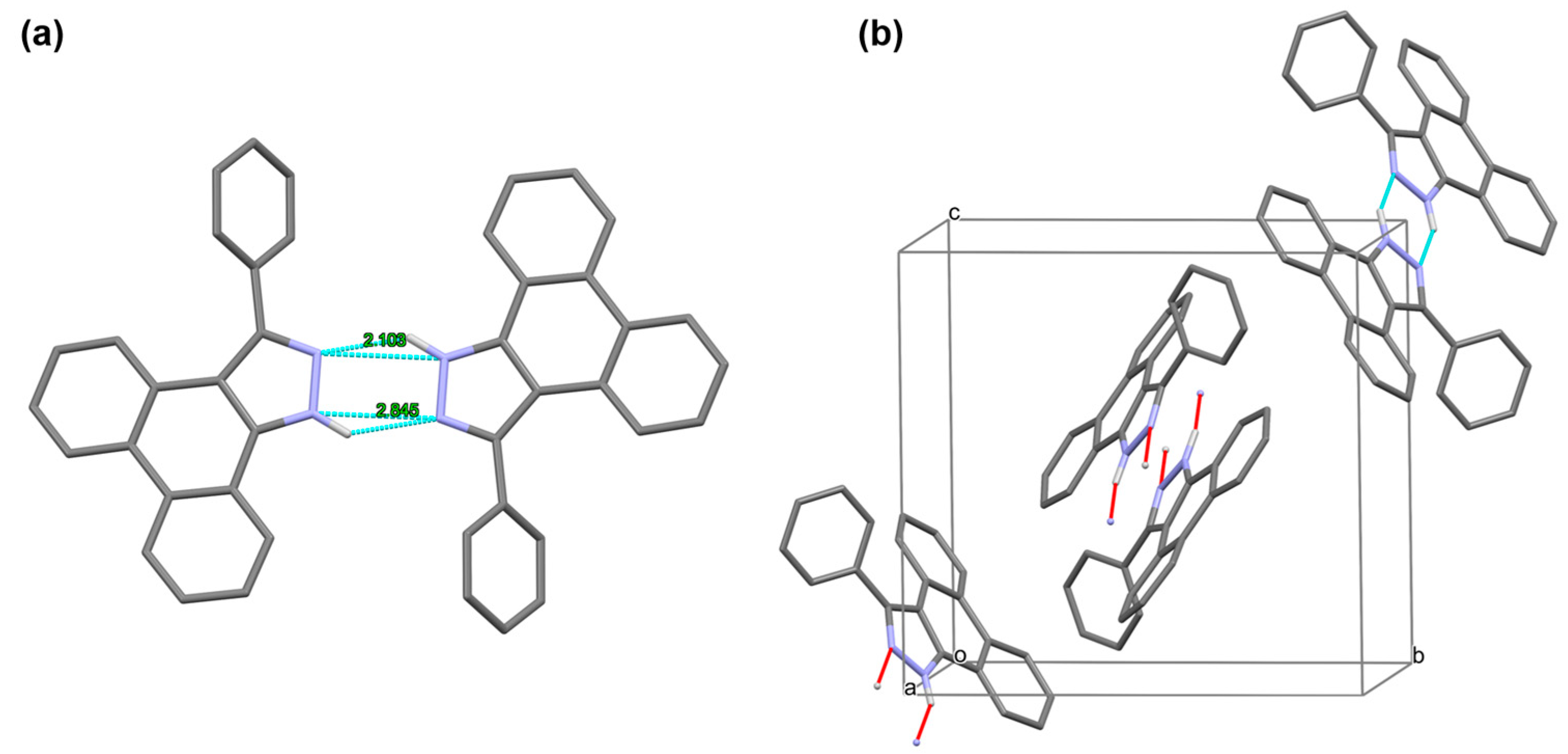The image depicts a complex and intriguing diagram with a white background, primarily featuring grey structures with colorful elements. It is divided into two sections labeled "A" and "B." 

In section A, on the left, the diagram showcases interconnected hexagon and pentagon wire shapes, reminiscent of chemical compositions or molecular diagrams. Dominating the center of this section is a larger hexagon with lavender and turquoise highlights. The top and bottom of this section display numbered measurements, "2.103" and "2.845," associated with turquoise colored lines.

Section B, on the right, features a 3D clear box with its corners labeled A, B, C, and O. Emerging from this box are helical chains, some appearing to link together, suggesting a dynamic, almost magnetic interaction. These chains also resemble wire structures forming hexagonal and pentagonal patterns, with some segments colored in lavender and turquoise. Of particular interest are bits that protrude from these chains, resembling red sticks capped with silver or lavender balls, possibly indicating points of connection or interaction.

Overall, the image, with its blend of detailed geometric patterns, vibrant color highlights, and scientific labeling, resembles an elaborate molecular model, offering a visually stimulating and intricate composition.